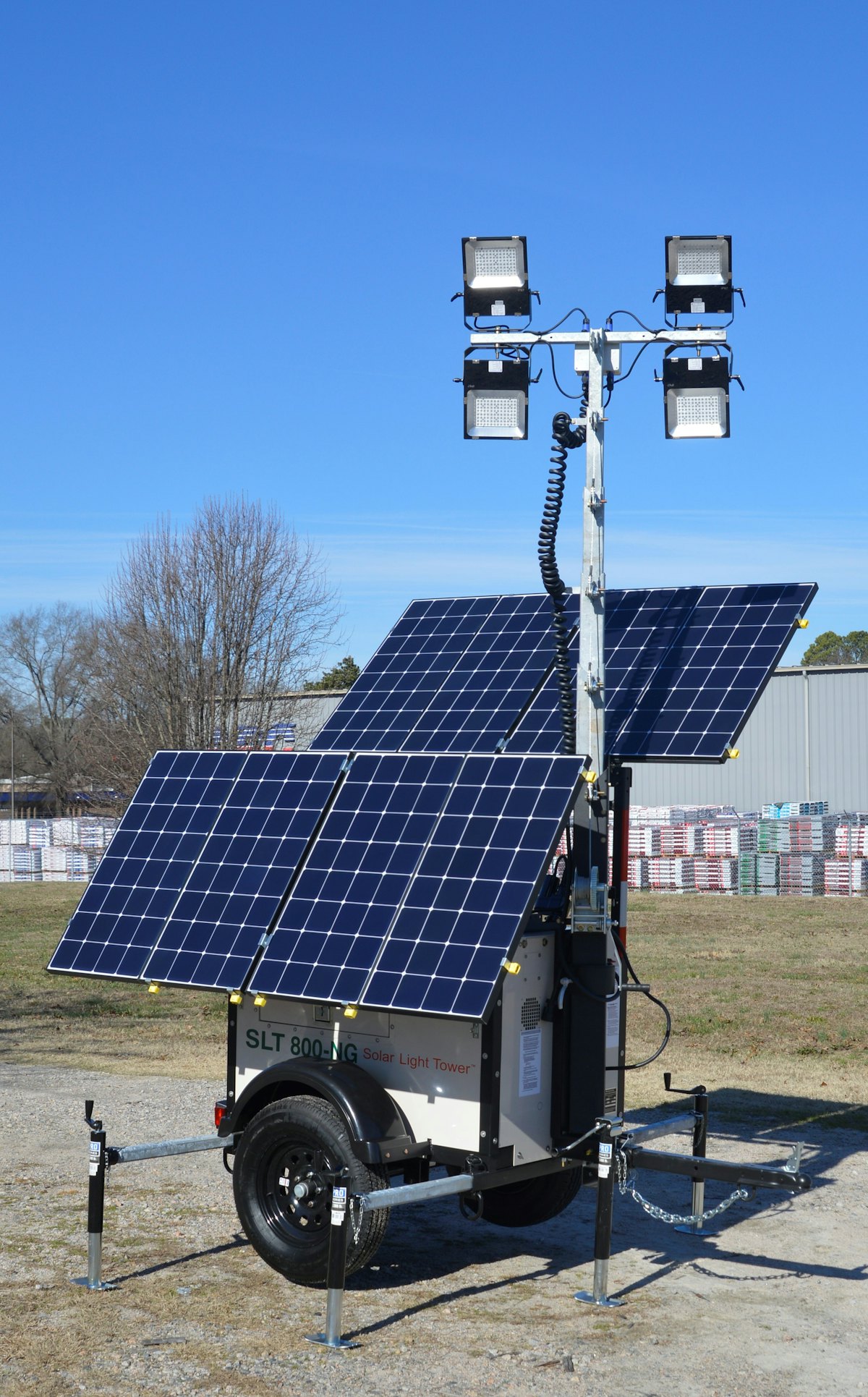In the image, there is a small trailer-mounted solar panel array with two large black solar panels angled toward the sun. The trailer is moveable, equipped with wheels, and features a prominent vertical pole topped with four lighting structures, two on each side. The trailer has green writing reading "SLT-800," accompanied by smaller, unreadable red text. The setup is situated on a gravel or dirt ground, amidst sparse patches of grass. In the background, a big gray warehouse is visible, with pallets or bags of soil stacked alongside it. Barren trees without leaves also appear, suggesting a winter setting. The sky above is a bright blue with a few long, wispy clouds, maintaining an otherwise clear day.